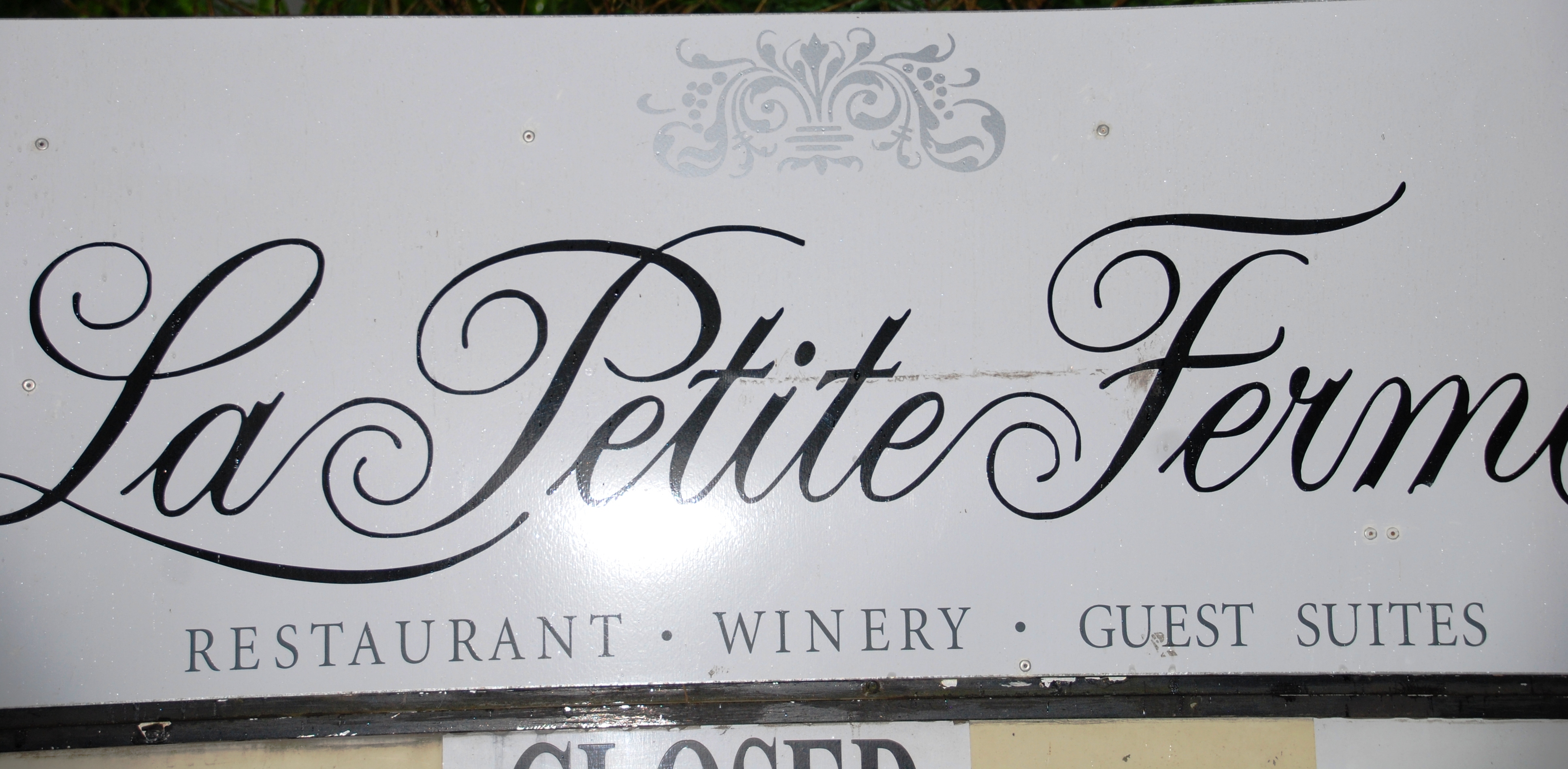The image showcases a photograph of a storefront sign positioned centrally within the frame, indicating a setting outdoors. Dominating the center, the sign features an elegant black cursive script spelling out "La Petite Femme Ferme Restaurant Winery and Guest Suites," though only "Ferme" and part of an "E" are fully visible due to the frame's crop. The sign itself is white with a black wooden border, adorned with a delicate floral pattern at the top. Beneath the cursive name, the words "restaurant.winery.guest suites" are clearly printed in black block letters. At the bottom edge of the image, a secondary sign with the word "Closed" in black font can be seen. The overall color palette of the image is defined by black, white, gray, and tan hues, with light reflecting subtly off the sign. The scene appears to be a closed restaurant's exterior, with part of the beige wall beneath the sign visible.